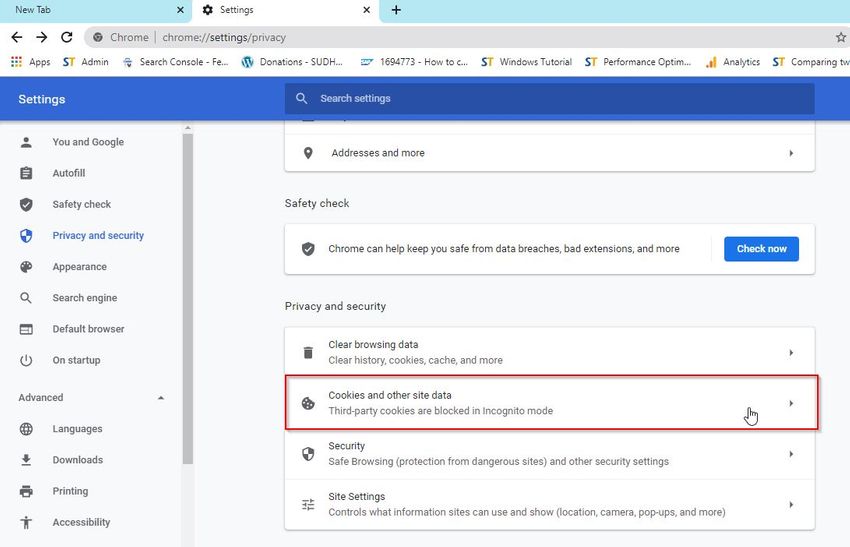**Descriptive Caption:**

The image depicts a slightly grainy and somewhat blurry screenshot of a web browser's settings page, taken within Google Chrome. At the top of the page, the screenshot shows a new tab on the left and the settings tab open on the right. The browser window has a white header, followed by a gray search bar displaying the URL "chrome://settings/privacy."

Below the URL bar, there is a bookmarks bar containing a series of bookmarked websites laid out from left to right: "Apps," "Admin," "Search Console," "Feed," "Donations," "SDDH (a WordPress site)," "1694773," "how to it," "Windows Tutorial," "Performance," "Optin...," "Analytics," and "Comparing."

Beneath the bookmarks bar, a blue horizontal bar spans the width of the page, labeled "Settings" on the left and featuring a search bar on the right with the placeholder text "Search Settings."

On the left-hand side of the page is a vertical navigation column with several sections listed from top to bottom: 
- "You and Google"
- "Autofill"
- "Safety Check"
- "Privacy and Security" (highlighted in blue)
- "Appearance"
- "Search Engine"
- "Default Browser on Startup."

Further down, under the "Advanced" section, additional options include:
- "Languages"
- "Downloads"
- "Printing"
- "Accessibility."

The central part of the page, which has a gray background, contains a prominent white box titled "Addresses and More." Directly below is another section called "Safety Check," including a message within a white box: "Chrome can help keep you safe from data breaches, bad extensions, and more." This section features a blue button labeled "Check Now."

Near the bottom of the screenshot, under the "Privacy and Security" heading, there is an option for "Clear Browsing Data," accompanied by text explaining the option to clear history, cookies, cache, and more.